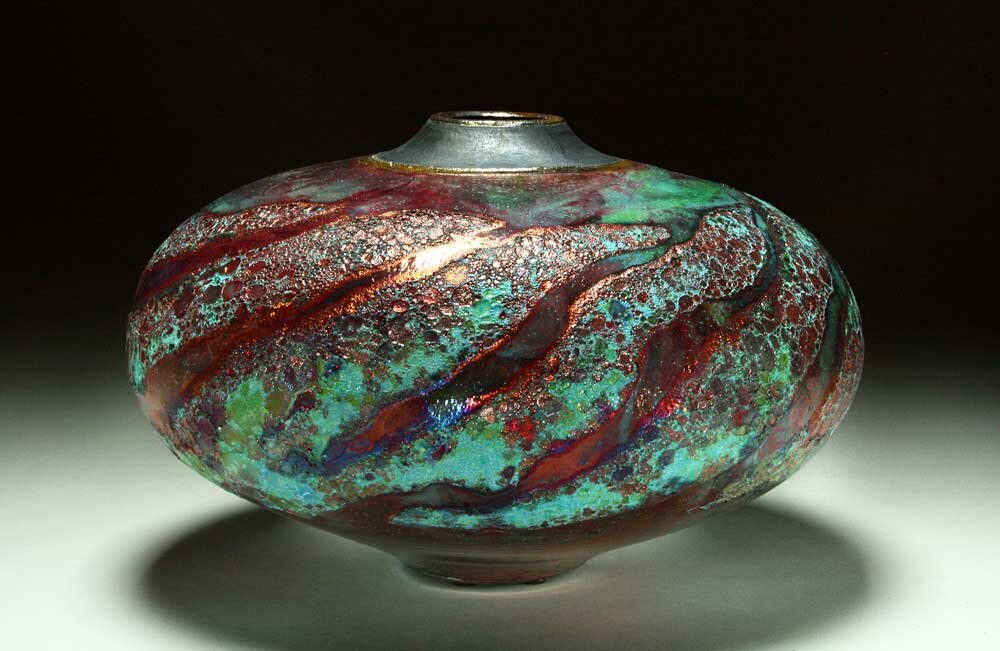This image is a very close-up photograph of a striking vase, likely taken in a museum setting. The backdrop is a solid black, enhancing the stark contrast with the white, shadowy surface on which the vase rests. This lighting setup directs attention to the vase, highlighting its details. The vase itself has a circular, elliptical shape that flares out towards the center with a small, round opening at the top and a narrow base. Its surface shimmers with a metal-like sheen, displaying a palette of turquoise blues, aqua greens, and dark reddish hues. Abstract red stripes run vertically, resembling scratch marks. The upper rim of the vase features a gold trim, adding an elegant touch. These elements together create an impression that is both vibrant and mysterious, as if the vase has been clawed at by some unseen force.